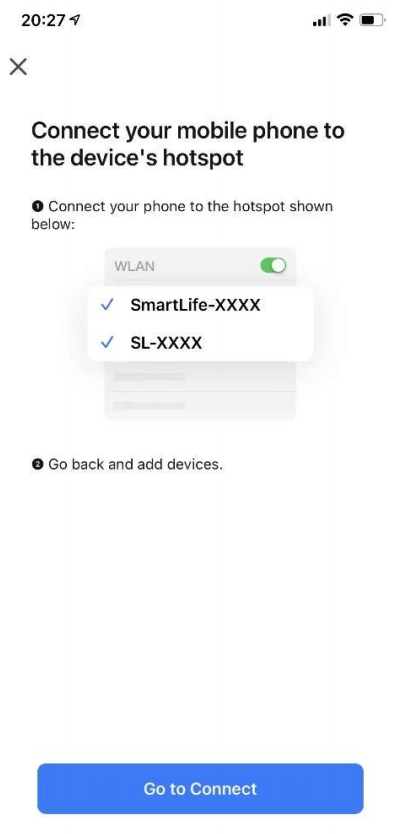The image appears to be a screenshot from an iPhone displaying instructions to connect the mobile phone to a device's hotspot. In the top-left corner, it shows the year "2027" alongside a location icon, and on the right, there are icons indicating signal strength, Wi-Fi connectivity, and a battery status at a bit more than half full. Just below this top banner, there's a gray 'X'.

The main section of the screen contains text that reads, "Connect your mobile phone to the device's hotspot." It details the steps as follows:

1. "Connect your phone to the hotspot shown below."
   
In this section, a toggle switch labeled "WLAN" is turned on. Below it, two blue check marks are present alongside network names "Smart Live - XXXX" and "SL - XXXX," indicating available hotspots. 

At the bottom, there is a blue button labeled "Go to connect."

Country-specific indicators suggest that the phone might be set to a European region, as indicated by the use of "WLAN" instead of "Wi-Fi" and the format of the time display. The screenshot also hints at the use of an app to facilitate this connection process.

Overall, the image provides step-by-step instructions for connecting to a device via a mobile hotspot.